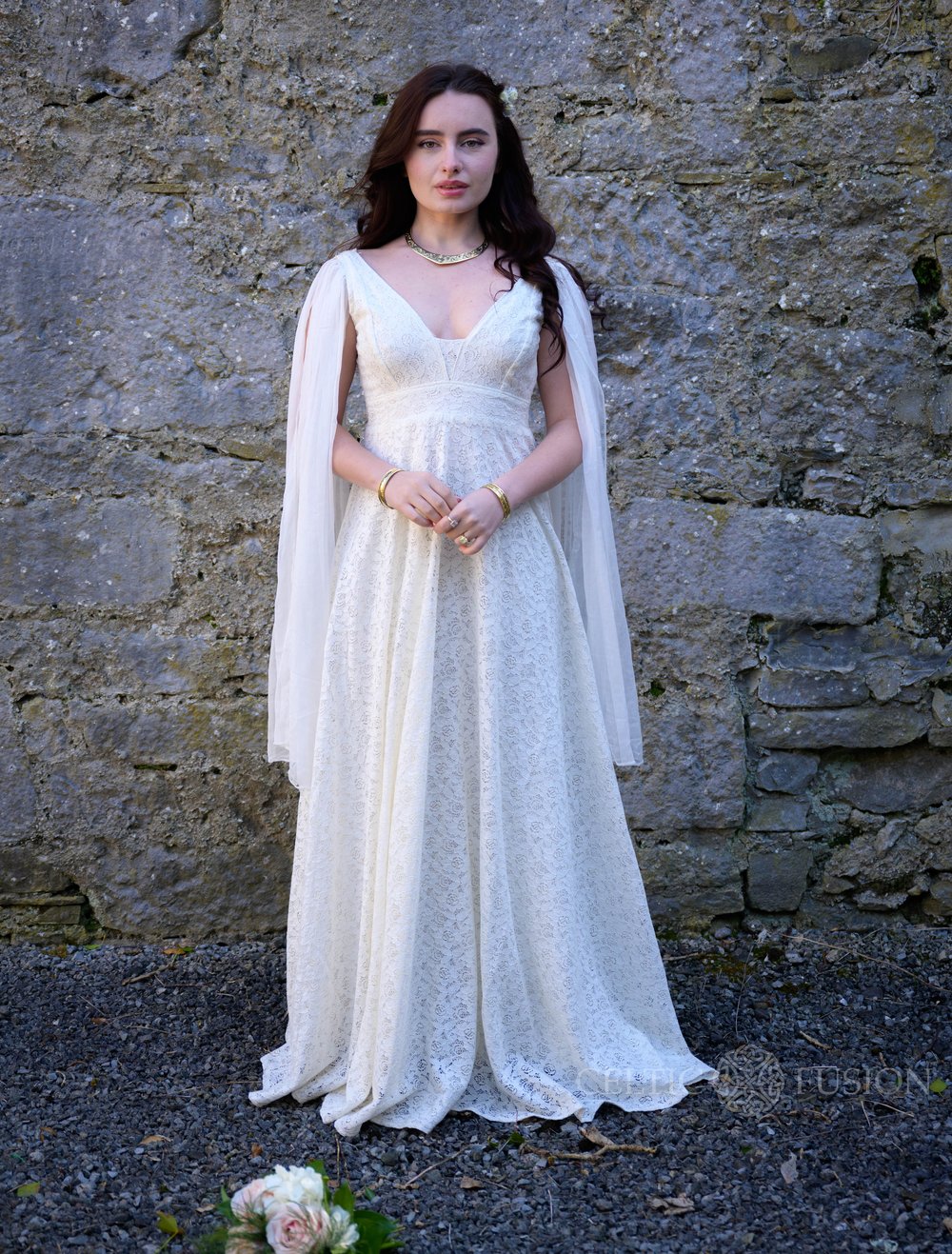This is a professional photograph of a young woman, possibly a bride or model, standing in front of an old, worn brick and stone wall. She is dressed in a floor-length, sleeveless white lace dress with a floral print and lacy trains that drape from each shoulder, partially covering her upper arms. The dress features a large V-neck, and she is adorned with gold jewelry, including a short gold necklace, a gold bracelet on each wrist, and a gold ring. The woman has pale skin, dark hair that falls to about shoulder length in loose waves, and dark eyebrows. She wears light makeup, including pink lipstick, and looks directly at the camera with her hands clasped in front of her stomach. At the lower edge of the photograph, a small plant with pink and white flowers and green leaves is visible. The ground is gravelly, and the bottom right corner of the image features a watermark with the partially illegible word "fusion" and a circular Celtic knot logo. This image exudes an artistic and elegant ambiance, suggestive of a wedding or a high-fashion photoshoot.